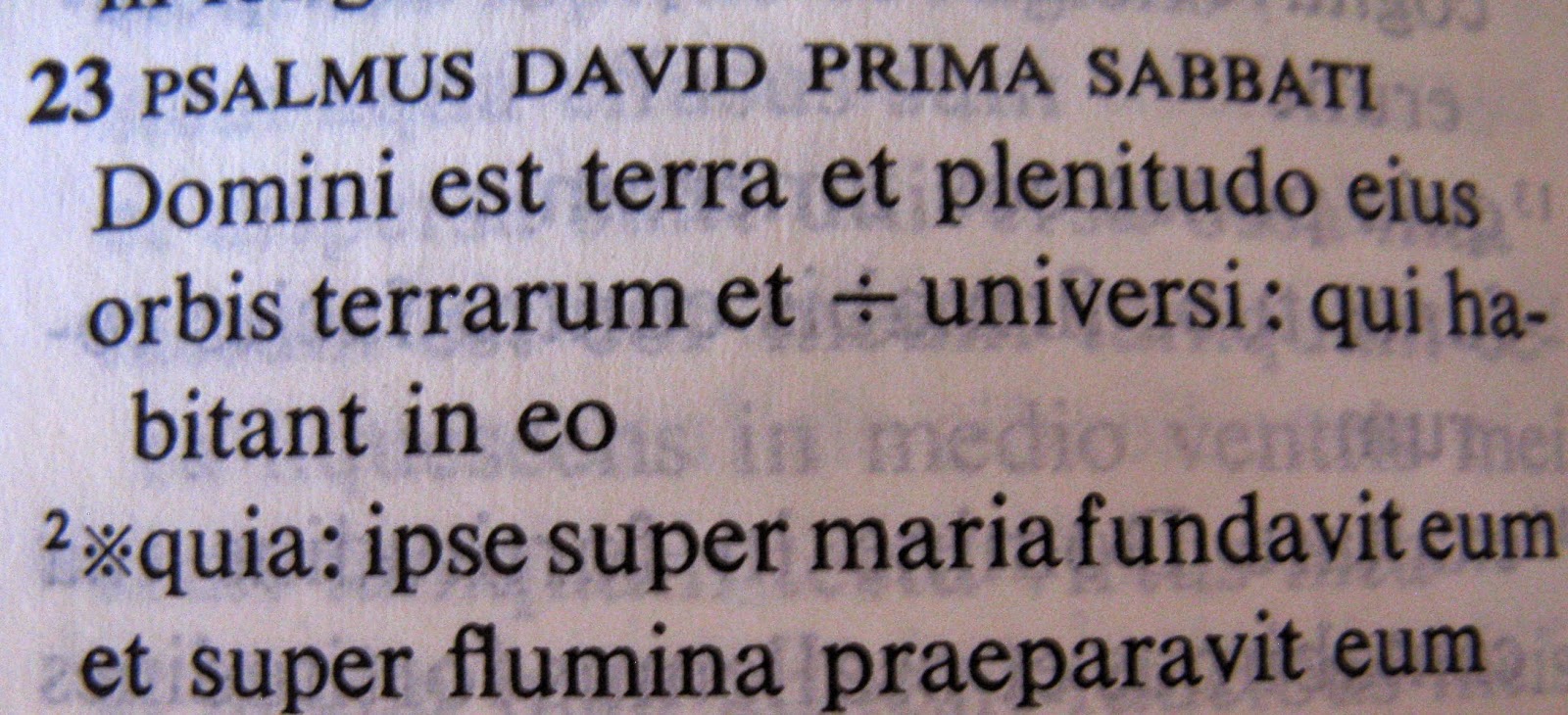This photograph captures a page from an old book, distinguished by its off-white, aged paper and black Latin text. The text on the page includes the word "psalmus," suggesting a connection to the Book of Psalms, as well as "David Prima Sabati," which might refer to a specific Psalm attributed to David and intended for a particular day. The top left-hand corner of the page is marked with the number "23," while the bottom left-hand corner features the number "2" alongside a unique symbol: an "X" surrounded by four dots. The meticulous details and classical elements of the typography suggest that this book holds historical or religious significance.